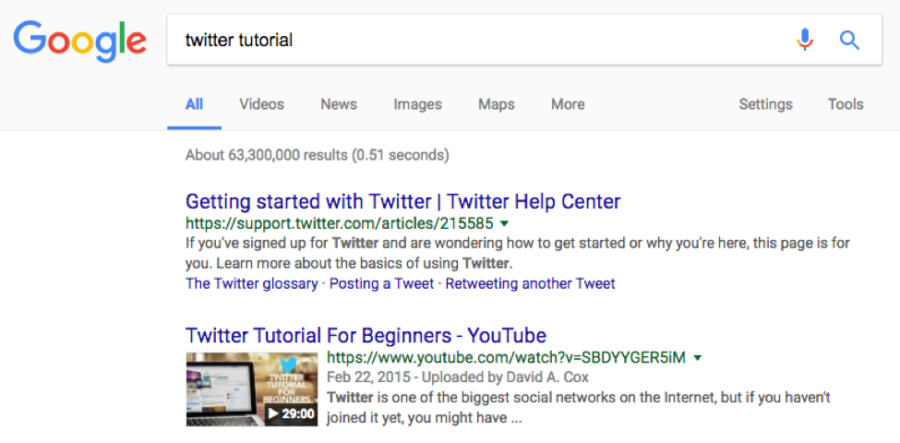The upper left corner of the image features the Google brand logo. Below that, in the search bar, the phrase "Twitter tutorial" is typed in black text. To the right of the search bar, there are a blue microphone icon and a blue magnifying glass icon.

Below the search bar, the word "All" is highlighted in blue and underlined, indicating the selected search category. Other available search categories include "Videos," "News," "Images," "Maps," "More," "Settings," and "Tools." The search results display "About 63,300,000 results" found in 0.51 seconds.

Highlighted in dark blue below the search statistics is a clickable link reading "Getting started with Twitter | Twitter Help Center." The URL for this link is "support.twitter.com/articles/215585."

The next section shows another result with a title in blue, "Twitter Tutorial for Beginners - YouTube." The associated URL, displayed in green, is "YouTube.com/watch." Beside this link is a square thumbnail image showing a computer screen and the iconic blue Twitter bird. The video has a total runtime of 29 minutes, indicated as "29:00."